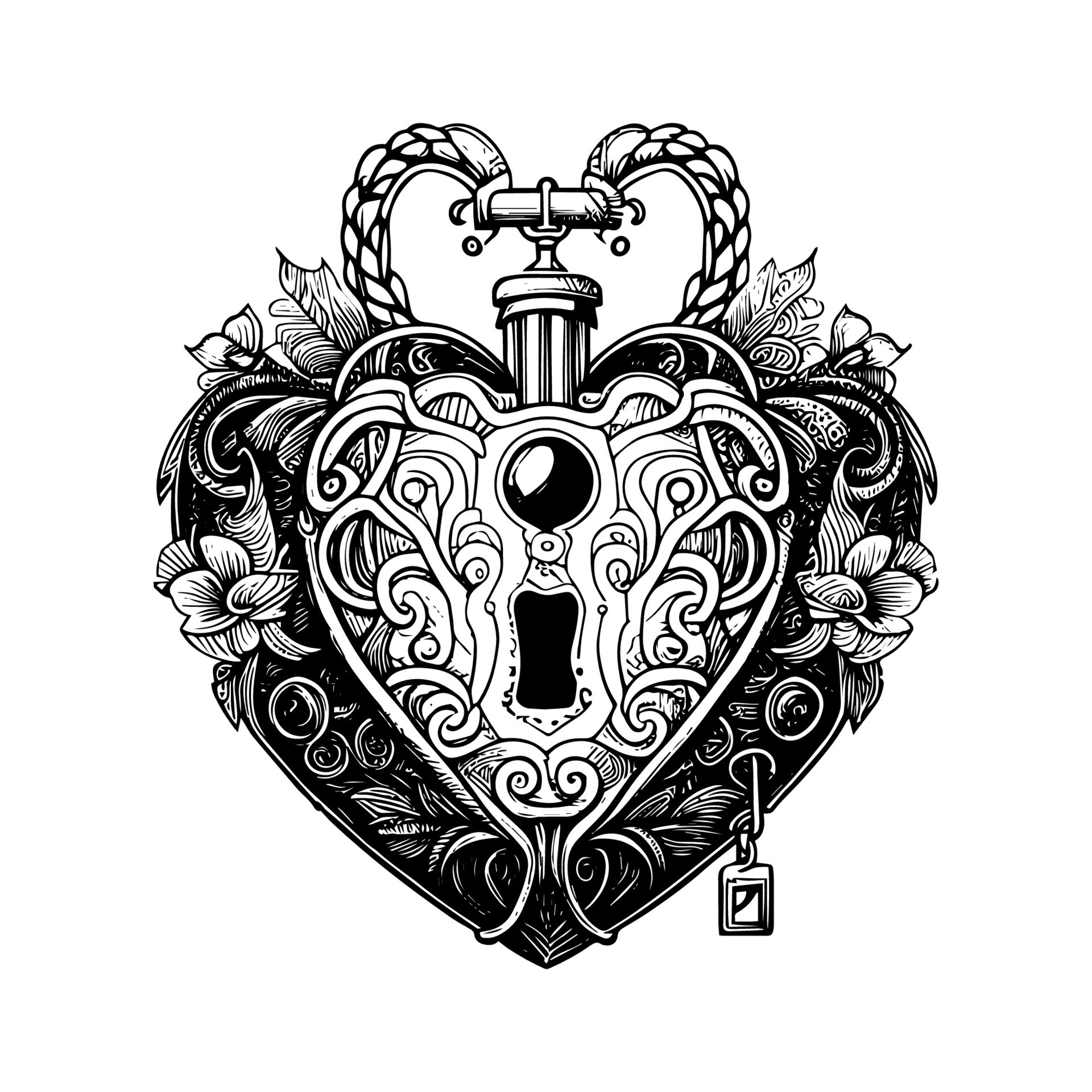This is a detailed black and white digital drawing of a heart-shaped locket. The locket features an intricate design primarily in shades of black, white, and gray. The main body of the locket is decorated with symmetrical, reflecting floral motifs and swirling patterns, giving it an elaborate, ornate appearance. The heart-shaped locket has a darker border with lighter tones in the center, enhancing its depth. The top handle of the locket is designed to look like a rope or string, allowing it to be hung, while a key hangs from the bottom part. The object is central in the image, with no accompanying text or artist signature, suggesting it could be clip art or a tattoo design. The overall image is highly detailed, highlighting the intricate decorations and floral patterns that adorn the locket.